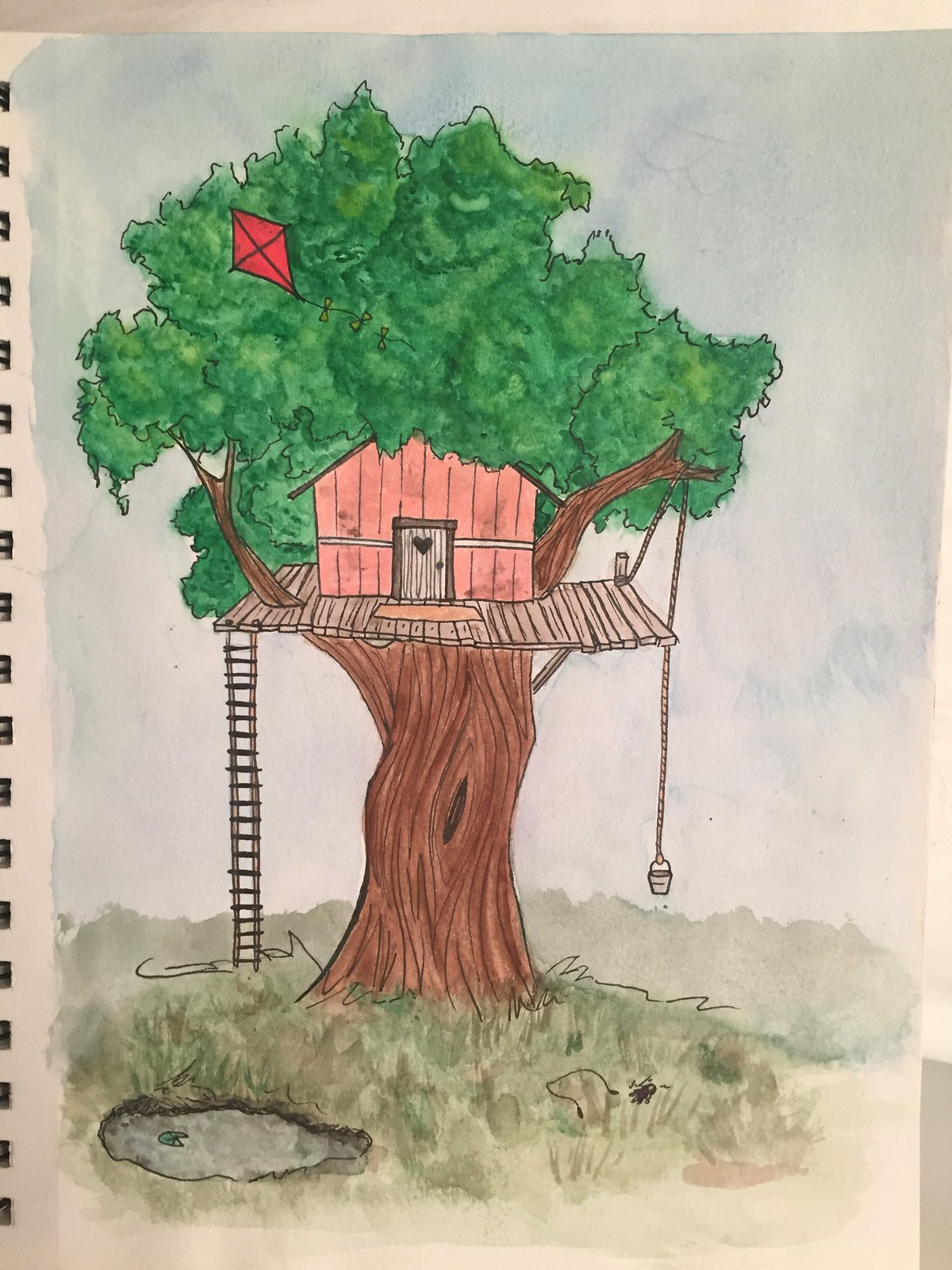In this beautifully detailed drawing on paper, hosted in a spiral-bound art book, a vibrant scene is depicted, seemingly painted with delicate strokes. Central to the artwork is a robust tree with a thick trunk, which features a small knothole partway up. Beneath the tree, a small puddle of water and patches of grass add a touch of nature to the scene.

Perched atop the tree is an enchanting treehouse, resembling a miniature wooden home. The treehouse sports a pointed roof and a charming door adorned with a heart-shaped cutout. In front of the door lies a welcoming mat, emphasizing the cozy feel of the tiny abode. Additionally, a ladder leads up to the treehouse, indicating a base built securely around the tree trunk.

Adding to the nostalgic allure, a kite is stuck in the upper branches of the tree, suggesting a playful, whimsical world. Completing the scene, a bucket hangs from a rope on one side of the treehouse, hinting at the practical, inventive nature of whoever might inhabit this delightful retreat.